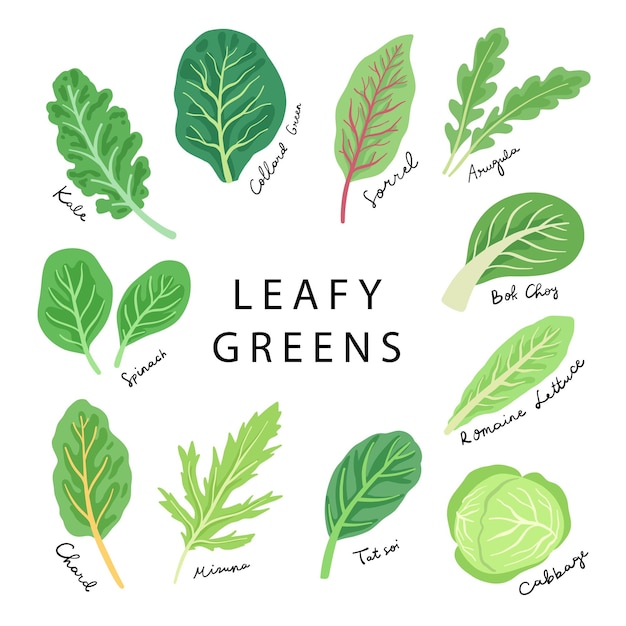The image is a digital or hand-drawn chart featuring various leafy green vegetables, set against a plain white background. In the center, bold black capitalized text reads "LEAFY GREENS." Surrounding this central text are cartoon-style drawings of individual leaves representing different types of leafy greens. These vector-drawn leaves, displayed in a circular pattern, are illustrated in a range of shades from light green to dark green, with some featuring yellow or purple hues.

Each leaf on the chart is accurately labeled with the name of the vegetable it represents, written in black cursive text positioned either below or to the side of the leaf. Starting from the upper left and moving clockwise, the leafy greens included are:

- A leaf labeled "Kale," featuring light green veins curving upwards and to the right.
- A wide, flat, dark green leaf with light veins labeled "Collard Green."
- A very light green leaf with a brown stem and veins labeled "Sorrel."
- Two dark green, narrow leaves with light green stems labeled "Arugula."
- A wide, flat green leaf with a wide stem labeled "Bok Choy."
- A light green, narrow leaf that tapers to a point, labeled "Romaine Lettuce."
- A round leaf with a light green color and darker outlines, labeled "Cabbage."
- A flat, dark green leaf with lighter veins labeled "Tat Soi."
- An oak-like light green leaf labeled "Minna."
- A flat green leaf with a long yellow stem labeled "Chard."
- Two flat green leaves with lighter veins labeled "Spinach."

This detailed chart not only visually differentiates each type of leafy green but also provides clear labeling for easy identification and educational purposes.